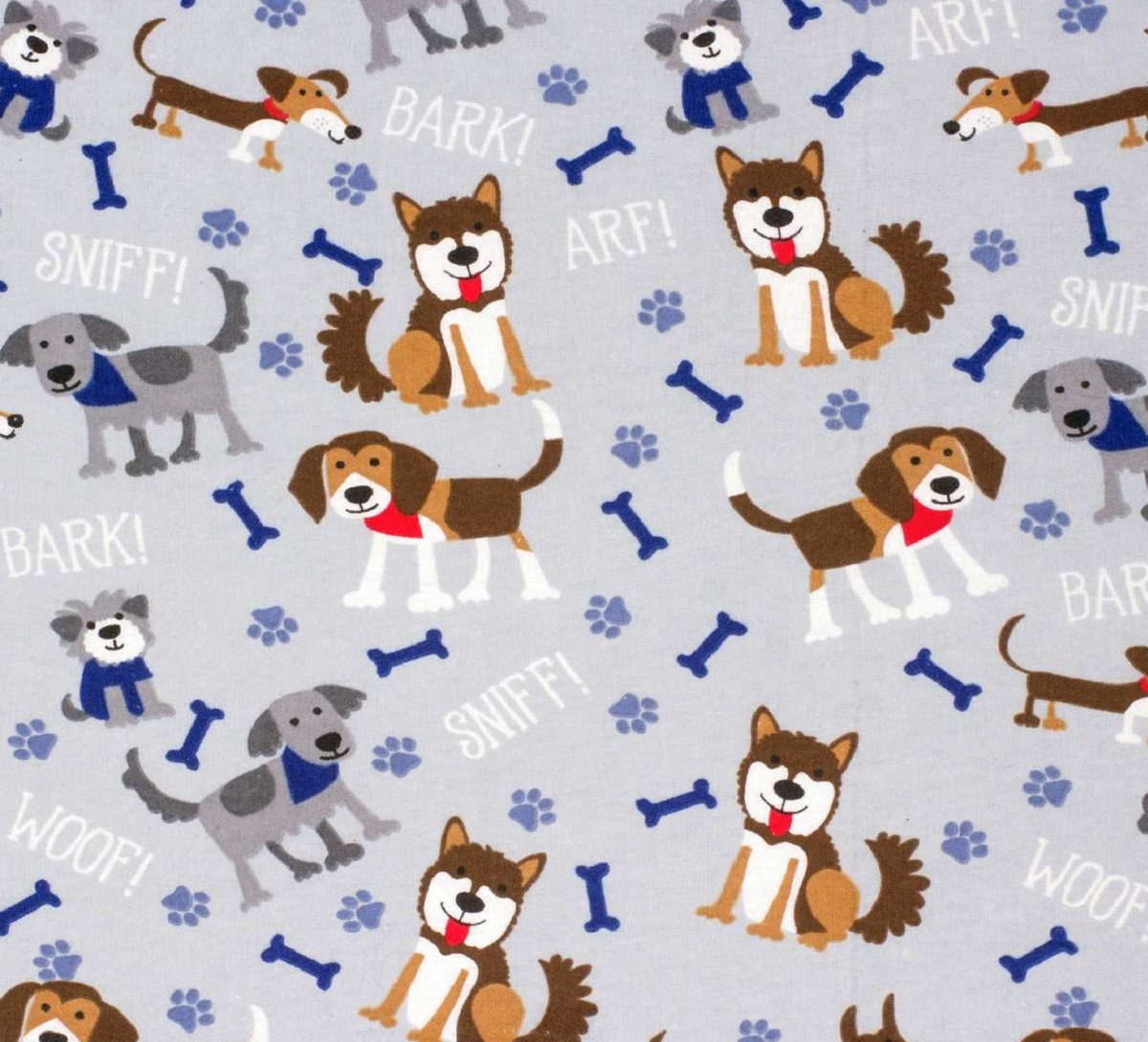The image is a detailed, square-format color illustration featuring a repeating pattern of various dog breeds. The background is a light blue-gray color, and the dogs are rendered in shades of brown and gray. One set of dogs has brown pointy ears, a red tongue sticking out, a dark brown tail, and a white chest and face. The other set has gray and dark gray fur with blue motif accents, such as a neck scarf. These dogs display different poses, with some sitting up and looking at the viewer and others standing in profile. Interspersed among the dogs are dark blue bones and light blue paw prints, along with white text reading "bark," "sniff," "arf," and "woof." The text appears at various angles, contributing to the whimsical and juvenile style of the illustration. The pattern resembles a textile print, such as might be found on soft fabrics like jersey or flannel, although no specific texture is discernible.